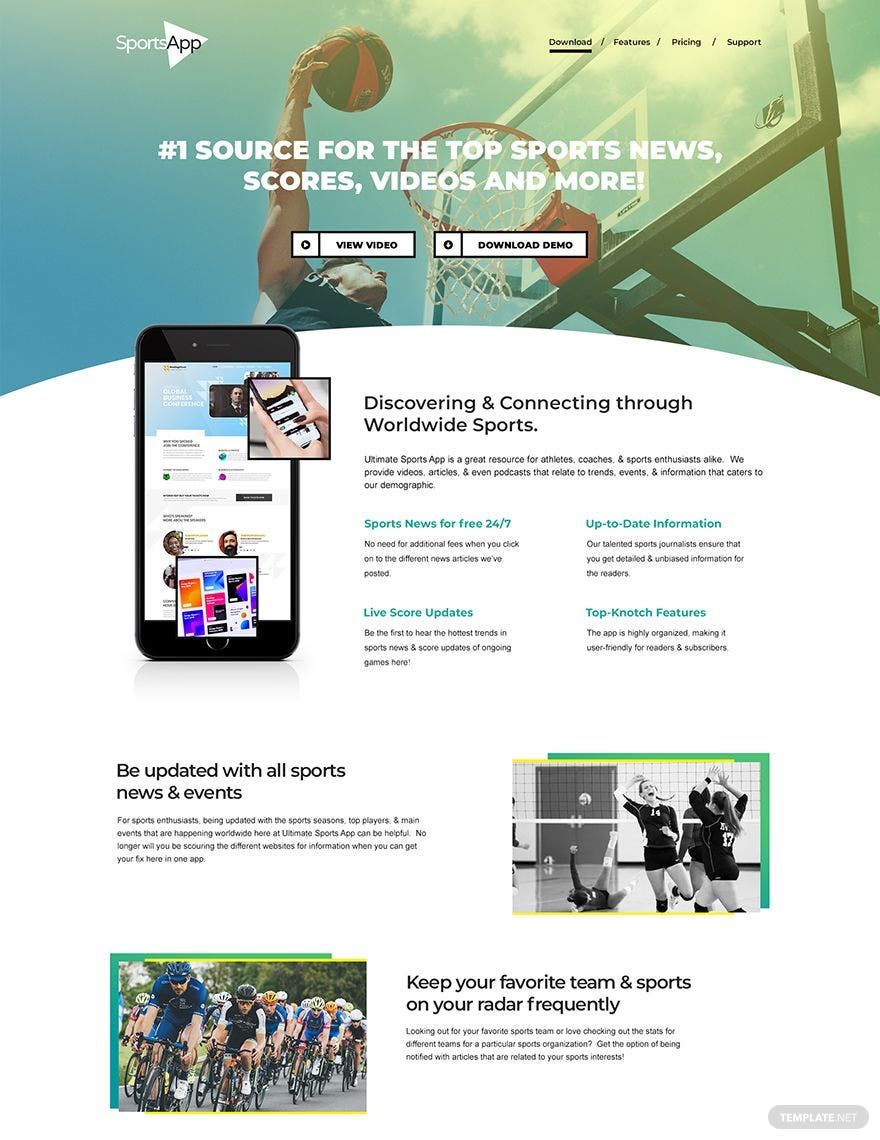The image is a screenshot of an advertisement for the "Sports App." The name "Sports App" appears in the top left corner, with "Sports" written in white and "App" in black within a sideways-facing triangle. The background shows an outdoor setting with a person mid-jump, either dunking a basketball or aiming to make a basket under a yellow-tinted color gradient.

To the right of the app name, there are four options in black font: Download, Features, Pricing, and Support. The center of the page prominently displays the tagline "The number one source for the top sports news, scores, videos, and more," in a bold white font. Below this, two white boxes contain options labeled "View Video" and "Download Demo," both in black font.

Further down, there is an image of a mobile phone with the app interface visible, showing someone scrolling through the app with their fingers. To the right of this image is a paragraph that highlights the app's ability to help users discover and connect through worldwide sports, detailing its features. Below this, a section encourages users to "Be updated with all sports news and events," providing more information about staying current with sports. The bottom right corner features another section emphasizing the app's ability to "Keep your favorite team and sports on your radar frequently," accompanied by various images of people engaging in different sports.